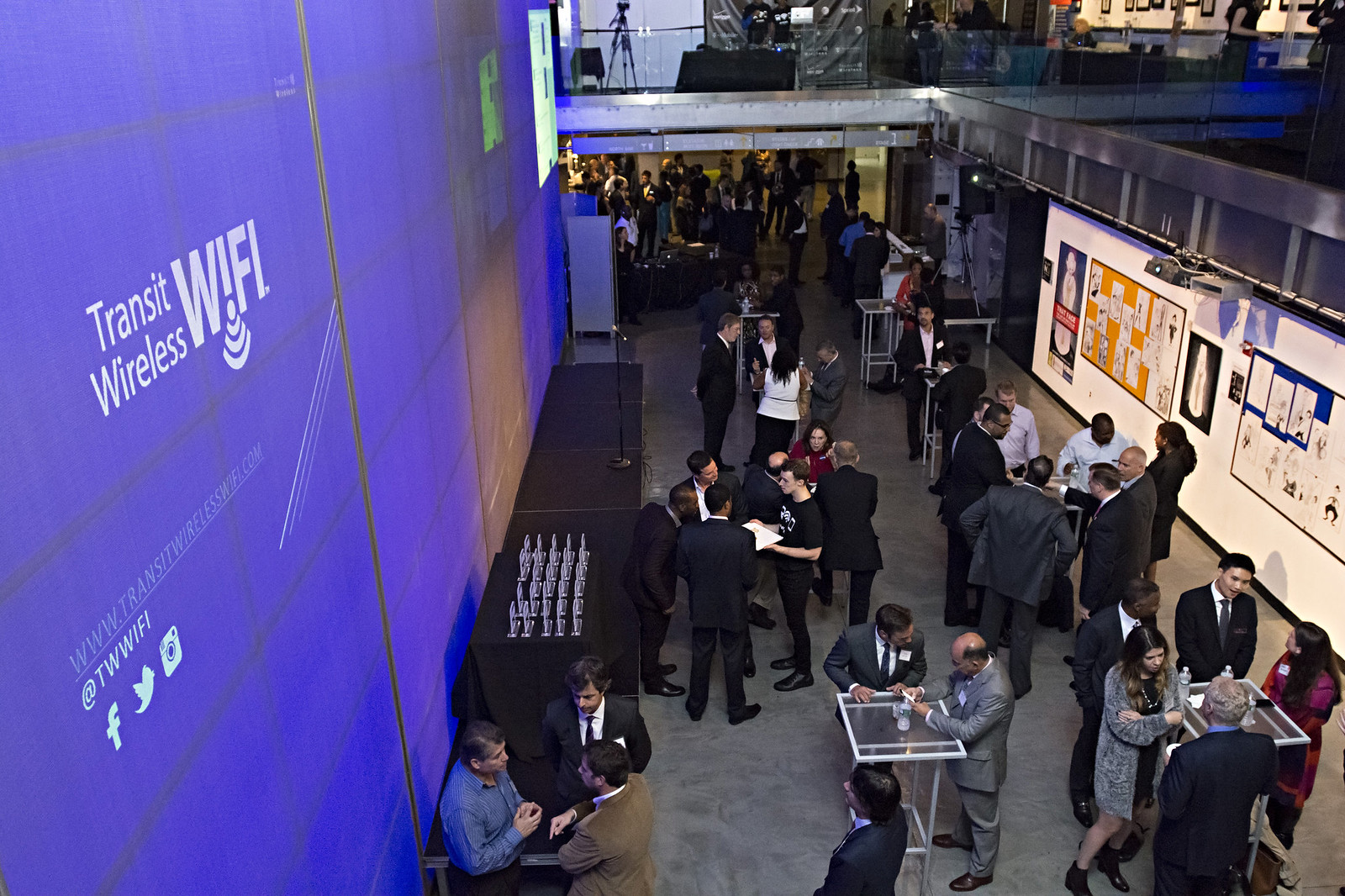The image captures a bustling tech fair or job fair with a vibrant, top-down view. The centerpiece is a large screen illuminated in purple, prominently displaying the logo and social media handle for Transit Wireless Wi-Fi. The venue is characterized by multiple floors and glass windows. Several tables, draped in black cloths, are scattered throughout the space, with at least one table having a glass top. Attendees in formal attire, predominantly men in suits, are engaged in conversations in small groups. Notably, three men in the bottom left corner are having a discussion; one in a blue shirt, another in a gray jacket, and the third in a black and white suit. The right side of the image features banners and drawings, while an orange and blue bulletin board are also visible. A whiteboard with various papers tacked on stands out, suggesting the presence of informational displays. The overall atmosphere is one of professional networking and engagement.